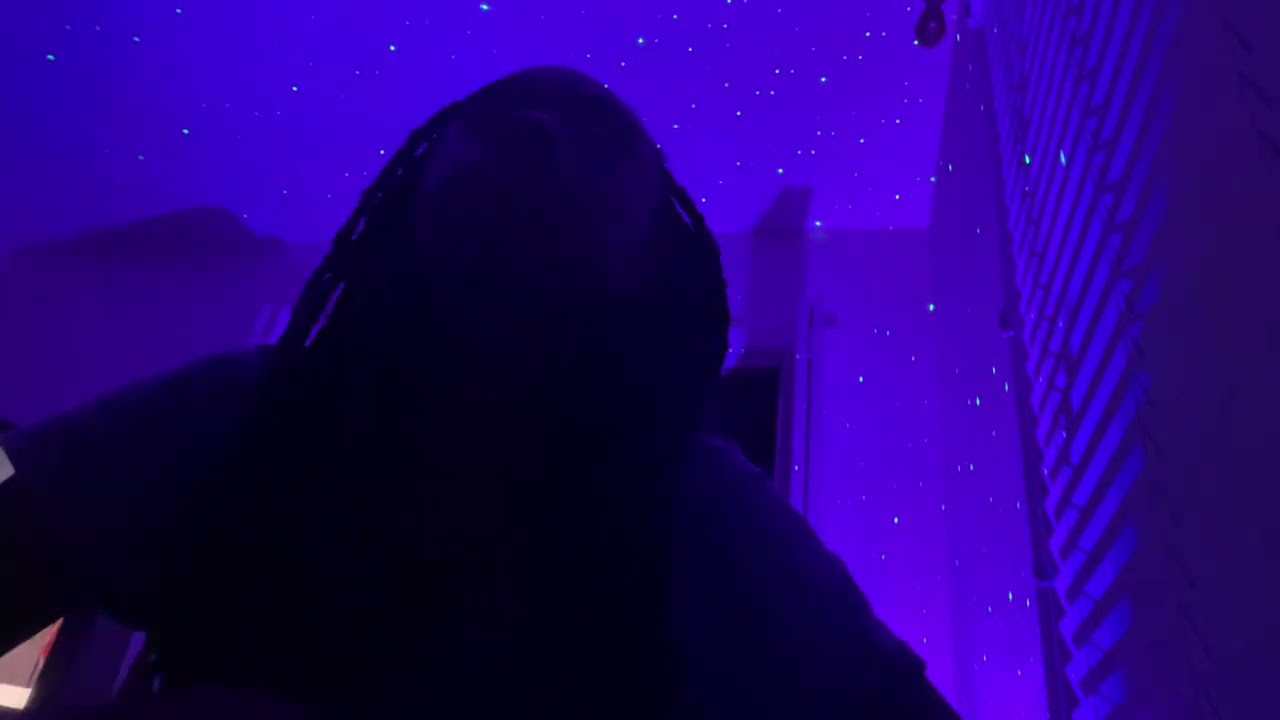A photograph shows a person from a low angle, making it appear that the photo is taken upwards from their waist toward their head. The person is difficult to discern as they are almost entirely cast in shadow, with only their hair being slightly visible; it seems they may have dreadlocks or long braids. The person is positioned on the left of the image, which is shaped like a widescreen TV.

In the background, the room is bathed in a vivid purple light with tiny white sparkles and star-like projections scattered across the walls, suggesting the use of a star projector. This ambiance creates an ethereal, almost surreal atmosphere. The room itself appears to be a bedroom or possibly an office, as suggested by a desk or the edge of a desk seen in the composition. On the right, there's a window with plastic curtains and blinds seemingly close to the person’s face, implying they are sitting near it. The room is devoid of conventional lighting, contributing to the overall darkness and enhancing the visibility of the star projections.